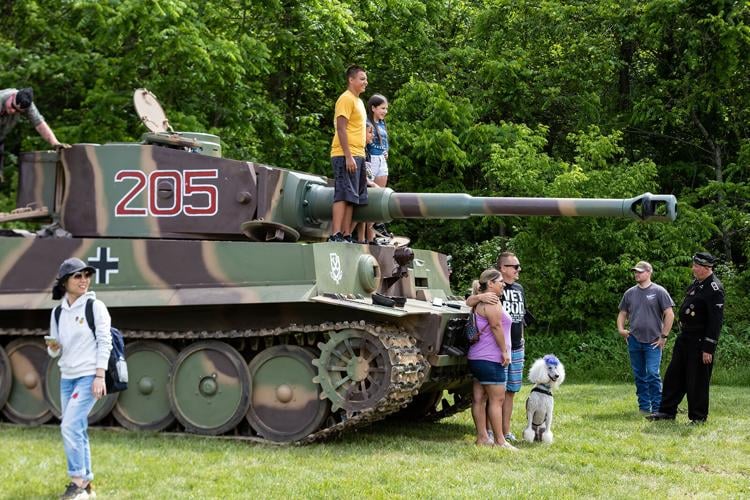This horizontally aligned rectangular picture depicts a vibrant outdoor scene on a sunny day, framed by a background of dense, leafy green trees. Prominently featured is an old military tank, camouflaged in olive green, beige, and brown, with the number "205" painted in red and outlined in white on its side. The tank, facing to the right, shows its cannon extending outwards and its circular track wheels visible below. Atop the tank, two young people—a boy and a girl—stand on either side of the barrel, posing cheerfully. 

In the foreground, on the left side of the tank, a woman in jeans, a white top, and a ball cap holds her phone, glancing sideways. Below the tank in the center, a man stands with his arm around a woman, accompanied by a white poodle at their feet. Nearby, a man in a black military uniform adorned with various insignias engages in conversation with another man dressed casually in a t-shirt and jeans, also wearing a ball cap. The entire scene is set on a lush green lawn, creating a striking juxtaposition between the vibrant natural surroundings and the historical military artifact.